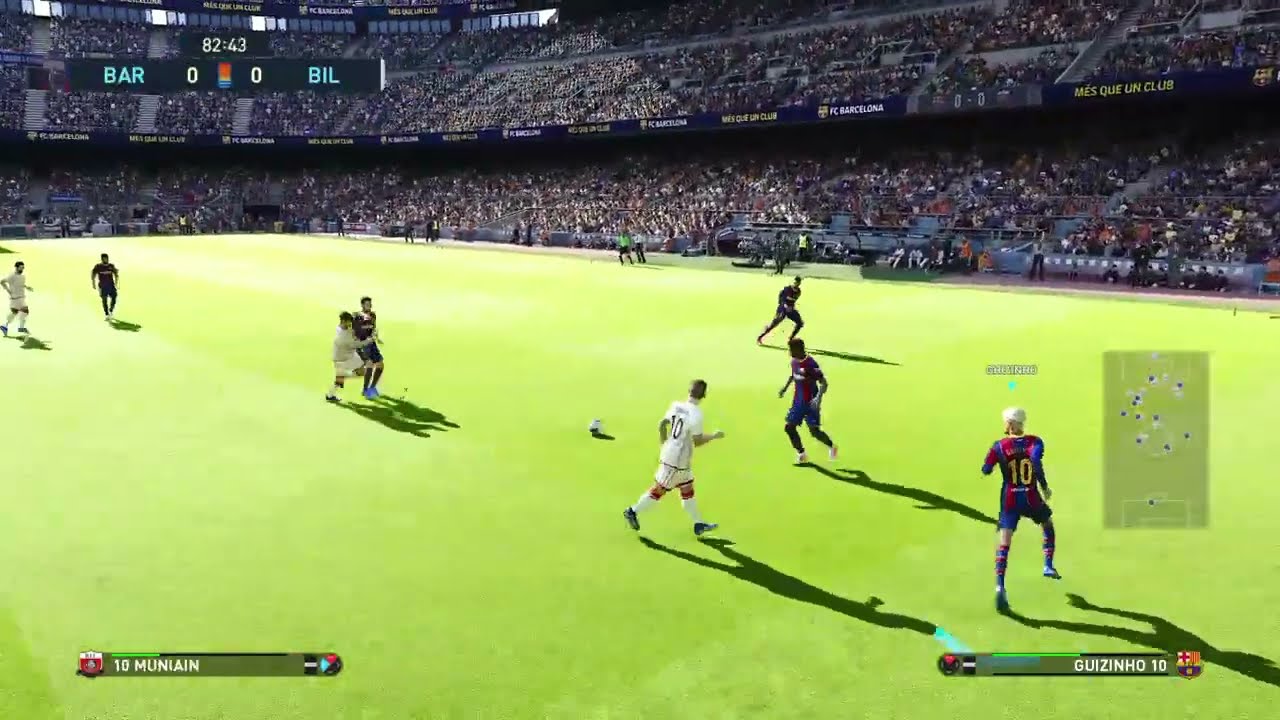The image appears to be a highly detailed and realistic screenshot from a soccer video game. It showcases a brightly lit, lime green football field with players actively engaged in the match. In the foreground, there is a soccer ball positioned slightly off-center, with a player in a white uniform standing just in front of it, while two other players collide nearby. To the right side of the ball, three players in blue and red uniforms can be seen.

In the background, an impressively packed stadium filled with two layers of fans stretches from the center left to the top right of the image. Along the stands, the words "Mesme Club" and an "FC Barcelona" badge can be observed, indicating the hosting team's identity. Overlapping the stadium view, at the top left corner of the screen, a digital scoreboard reads 82:43 in white, with team abbreviations "BAR" and "BIL" both showing a score of zero. There are various graphics overlaying the image, including rectangular indicators in white and blue, as well as a small map in the lower right corner depicting player positions on the field with blue dots.

Additionally, player names and numbers are displayed on the bottom corners of the screen: "10 Moonean" on the left, possibly with a flag symbol, and "Cusino 10" on the right. This intricate depiction suggests not only the intensity of the match but also the meticulous design of the game, bringing an immersive soccer experience to the viewer.